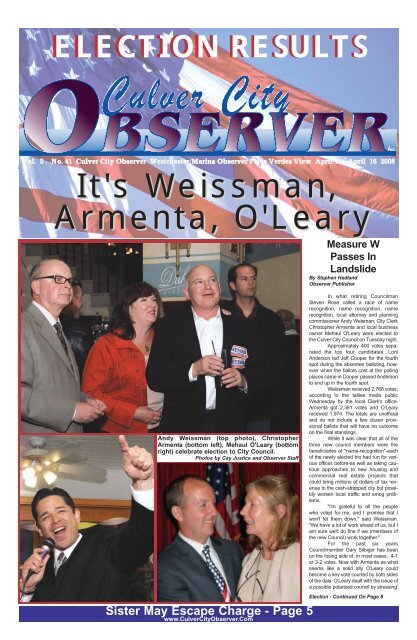This vertical rectangular image is a photograph of a local newspaper cover, specifically the Culver City Observer's edition announcing election results. At the very top is a background of a flag in lighter colors, overlaid with the headline "Election Results" in bold white letters. Beneath this, the newspaper's name, "Culver City Observer," is prominently displayed, with "City" in a lighter shade of blue and "Observer" in dark blue letters. The date "April 16, 2008" is also visible.

Below the masthead, the names "Weissman, Armenta, O'Leary" are presented in blue letters against the flag background, identifying the winners of the local election. Accompanying this text are photographs of the election victors. The images feature a man in a tan suit, a woman in a red jacket, a man in a black suit, and another individual in a black shirt. They appear to be looking up at something, possibly a screen.

Further down, there are additional images: one of a man in a black suit with a microphone, and another photo showing a man and a woman closely interacting. The man is wearing a gray suit with a red, white, and blue tie, smiling at a woman in a tan suit. Below these pictures, headlines include "Sister May Escape Charge Page Five" and the website "www.culvercityobserver.com," alongside details about the election results.

A column of text on the right side of the image reports, "Measure W Passes in Landslide," providing further context and detailed results of the election.